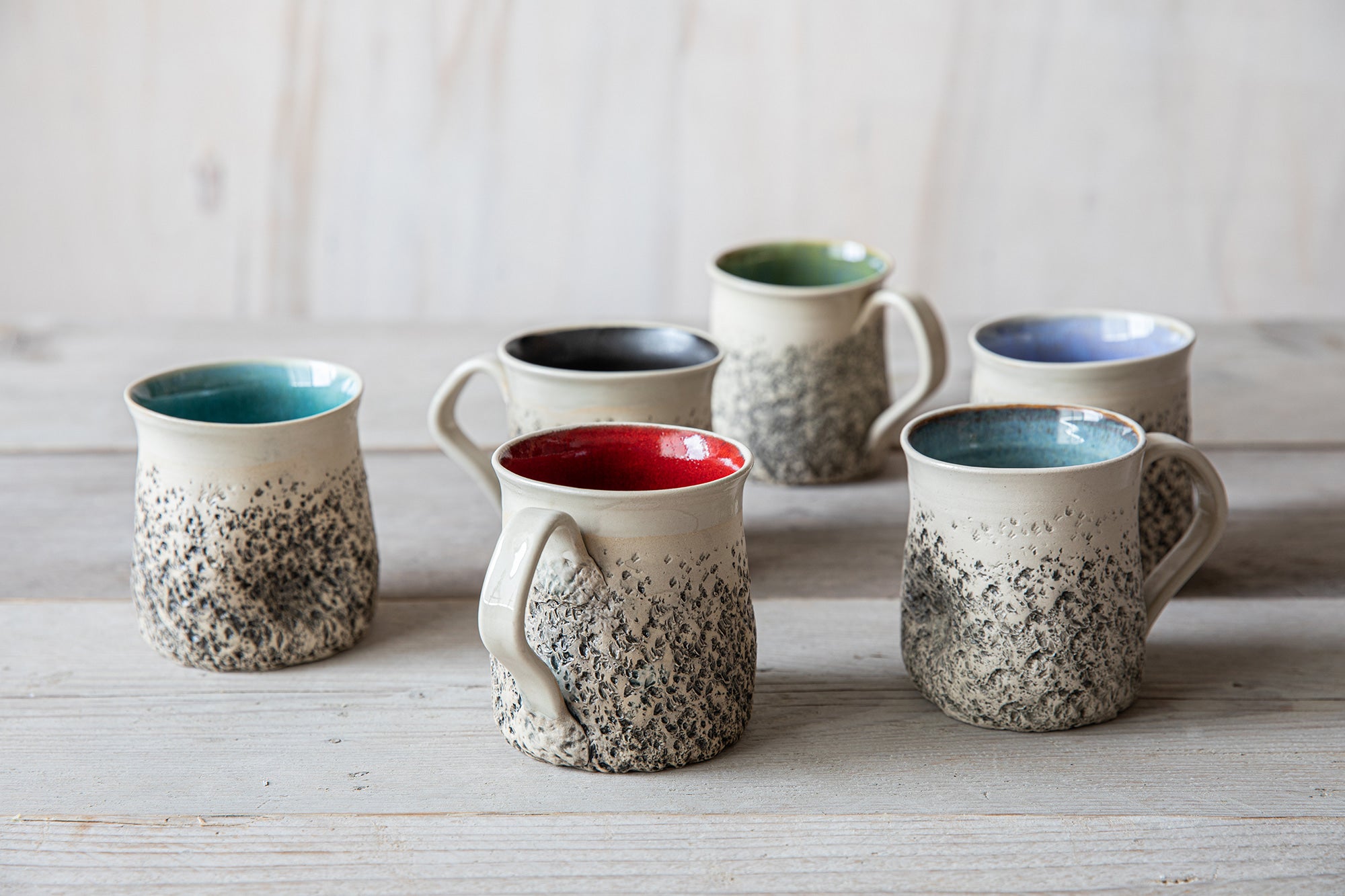This detailed photograph captures six handmade ceramic mugs arranged on a rustic, white-painted wooden table set against an out-of-focus matching background. The artisanal mugs, each one unique yet collectively cohesive in style, exhibit a cream-colored exterior with black stippling on the lower two-thirds, resembling a textured, handcrafted finish that becomes smoother towards the top. Their interiors are vibrantly glossy, featuring a diverse palette of colors that range from teal, red, and dark blue to green, light blue, and lavender. The composition evokes a French country aesthetic, enhanced by the table's charming patina and the subtly shadowed arrangement of the mugs, which adds depth and visual interest to the image.